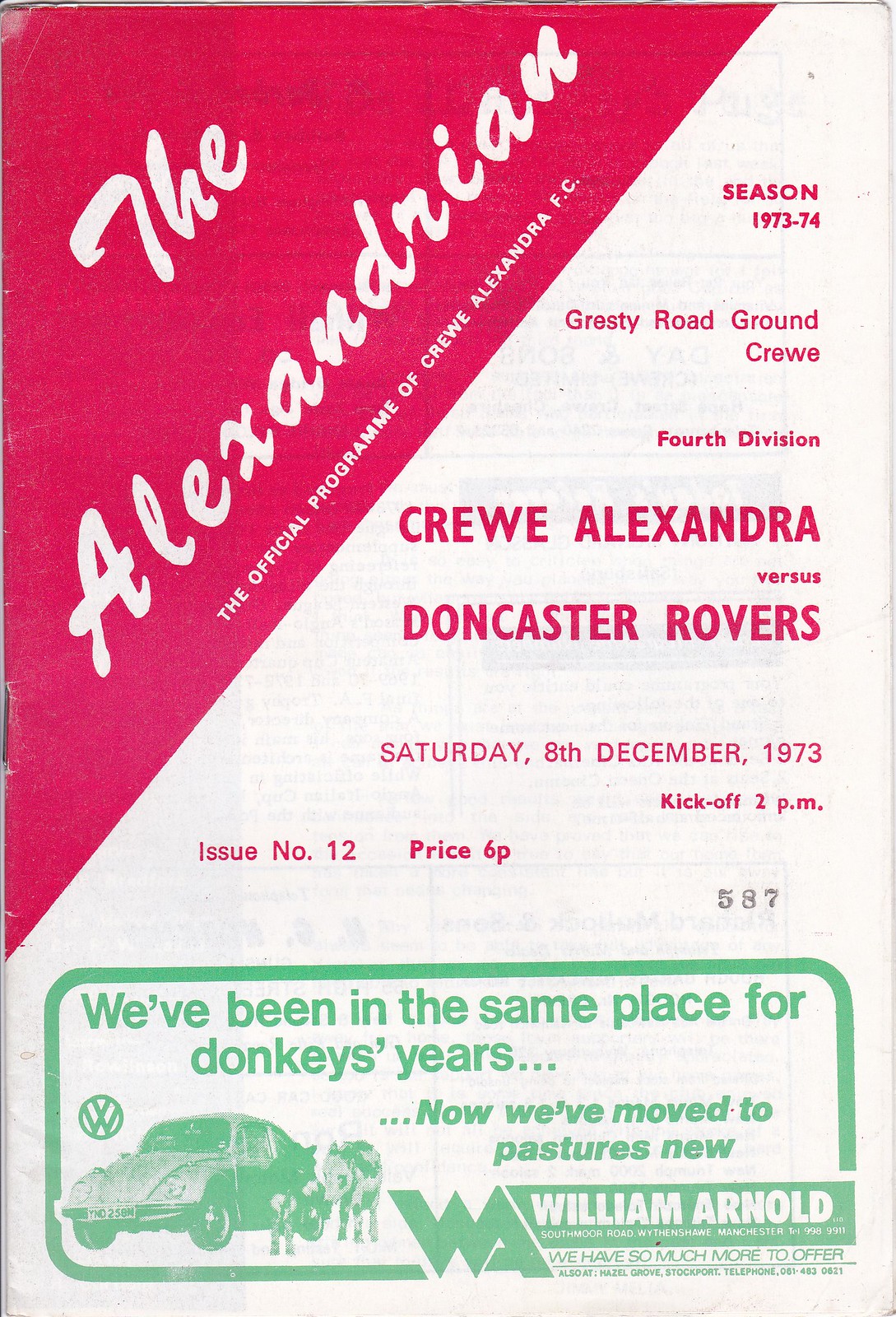The image depicts the front cover of a football program for Crewe Alexandra FC from the 1973-74 season. Dominating the upper left corner, a red triangle with white text announces "The Alexandrian," identifying it as the official program of Crewe Alexandra FC. Adjacent, in the upper right corner, white text on a red background indicates the season (1973-74), while below, details like "Grady Road Ground Crew" and "4th Division" are mentioned. Highlighting a specific match, bold red letters state "Crewe Alexandra vs. Doncaster Rovers, Saturday, 8th December 1973, kickoff 3 p.m." Additionally, the issue number (12) and the price (6 pence) are specified. The bottom part of the page features an advertisement bordered in green, depicting a Volkswagen with the VW emblem, two donkeys next to it, and text that humorously remarks on the dealership's long-standing location, now relocated. The ad includes "William Arnold" and "WA," suggesting the dealership's name. The cover's color scheme includes black, pink, white, green, and grey, enhancing its vintage style.